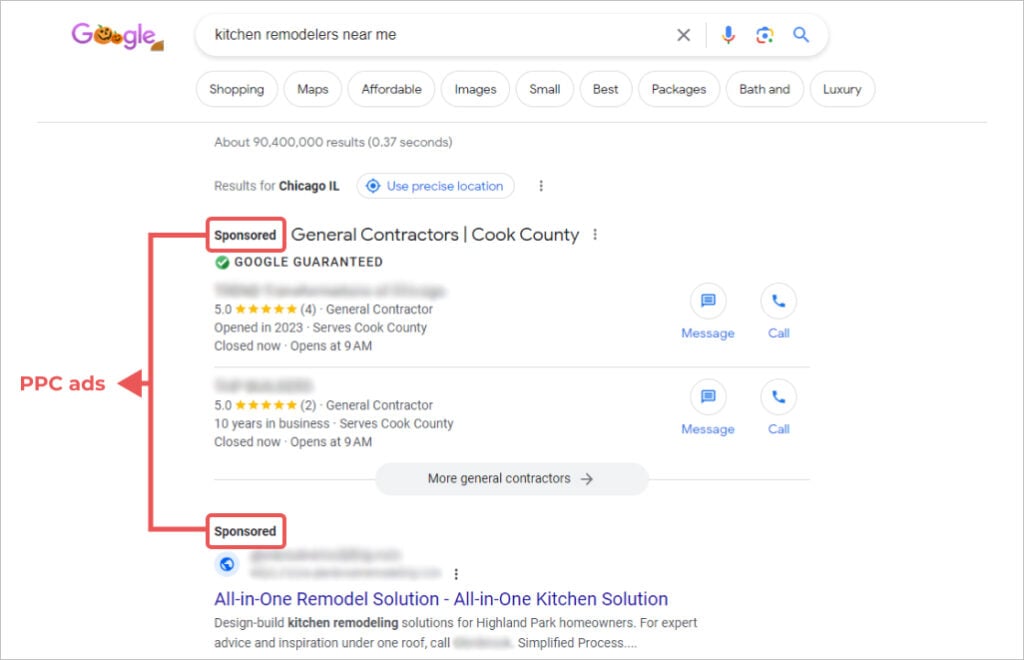On Halloween, a festive Google search is displayed, featuring the Google logo in a Halloween theme: a traditional red G, two pumpkins for the O's, followed by 'G L E' in purple. The white oval search box, where "kitchen remodelers" has been typed in black, stands out beneath the logo. Below the search box are several clickable ovals, white inside with gray outlines, each labeled in black text, reading: "shopping," "maps," "affordable," "images," "small," "baths," "packages," "bath," and "luxury." A thin gray line stretches across the screen, beneath which it states there are about 90,400,000 results in 0.37 seconds, specifically targeting Chicago, Illinois. 

A blue link offers to "use precise location" next to the text "results for Chicago, Illinois." A pair of "sponsored" results is identified in small boxes, connected by lines to red text reading "PPC ads" along with a red arrow. The first sponsored result is for "General Contractors," guaranteed by Google with a blurred address, five-star rating from four reviews, stating they serve Cook County, open at 9 a.m. in 2023 but currently closed. The bottom text includes a blue link for an "all-in-one remodel solution" and "all-in-one kitchen solution."